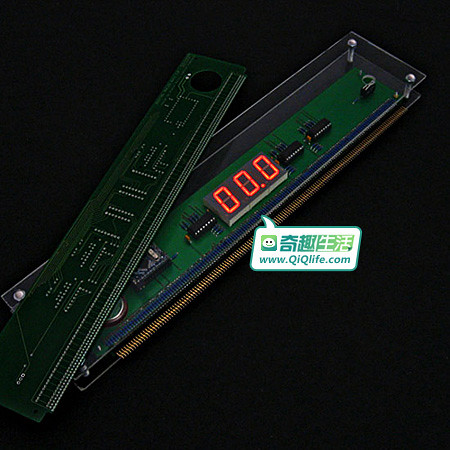This detailed color photograph features a green rectangular circuit board, suggestive of a computer component like RAM, prominently displayed diagonally from the lower left to the upper right corner. This circuit board, fitted with sockets for integrated circuits, sits atop a piece of rectangular plexiglass, which overlays another green printed circuit board below. The lower circuit board contains three or four integrated circuits and a central, illuminated three-digit LED display showing all zeros. Accompanying this display is a white rectangular overlay with green Asian characters and the URL "www.qiqlife.com". The background of the image is entirely black, enhancing the visibility of the components.